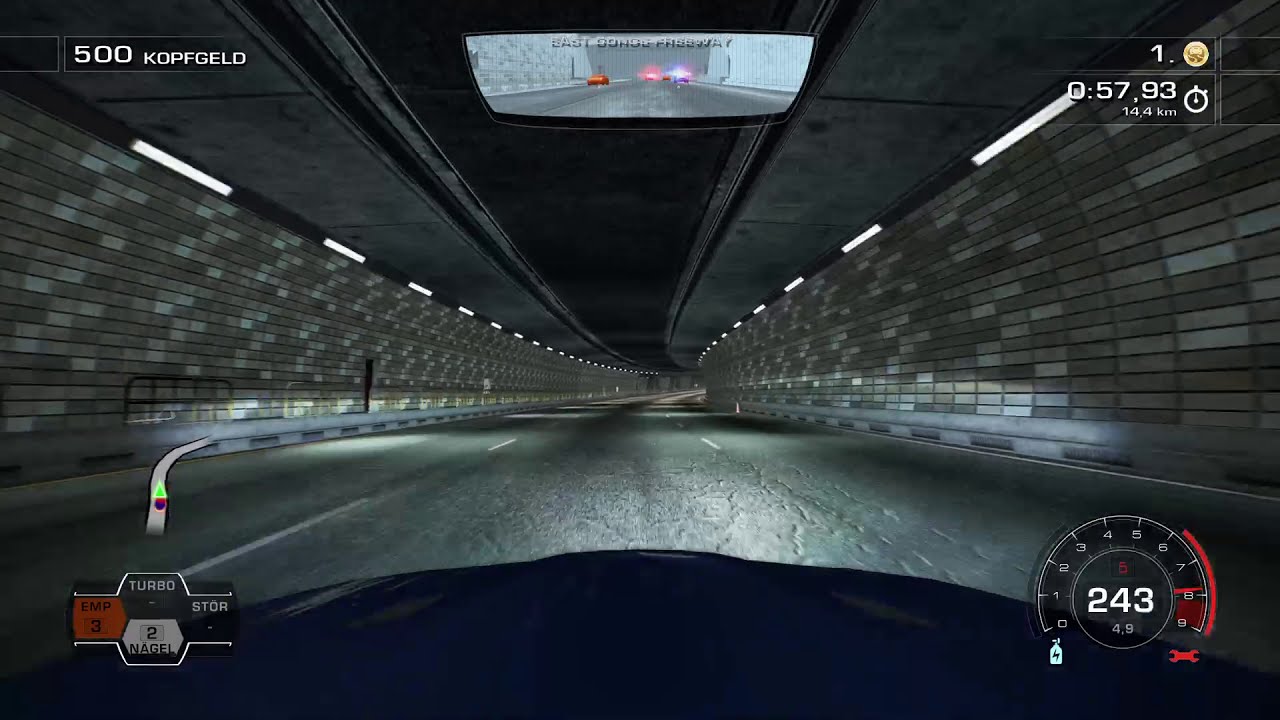This is a detailed screenshot from a video game featuring a first-person view inside a blue car driving through a dimly lit underground tunnel with stone brick walls. The tunnel's ceiling is lined with white tube lights, casting a glow over the scene. Both sides of the road are paved and bordered by brown rectangular bricks. Visible through the car's rear-view mirror are flashing red and blue police lights, suggesting a high-speed chase. In the lower-left corner, a map displays the road ahead, along with various controls labeled Turbo, EMP, NAGEL, and STOR. An orange square and white detail are also on the map display. The bottom right corner features a speedometer reading "243," while the top right corner shows a distance counter at "14.4 KM" and the current time. The top left corner displays the text "500 Kopf Geld." The center of the screen shows the road through the tunnel and the hood of the car, immersing you in the driving action. The predominant colors include gray, black, red, blue, and gold, contributing to the racing game's intense and focused atmosphere.